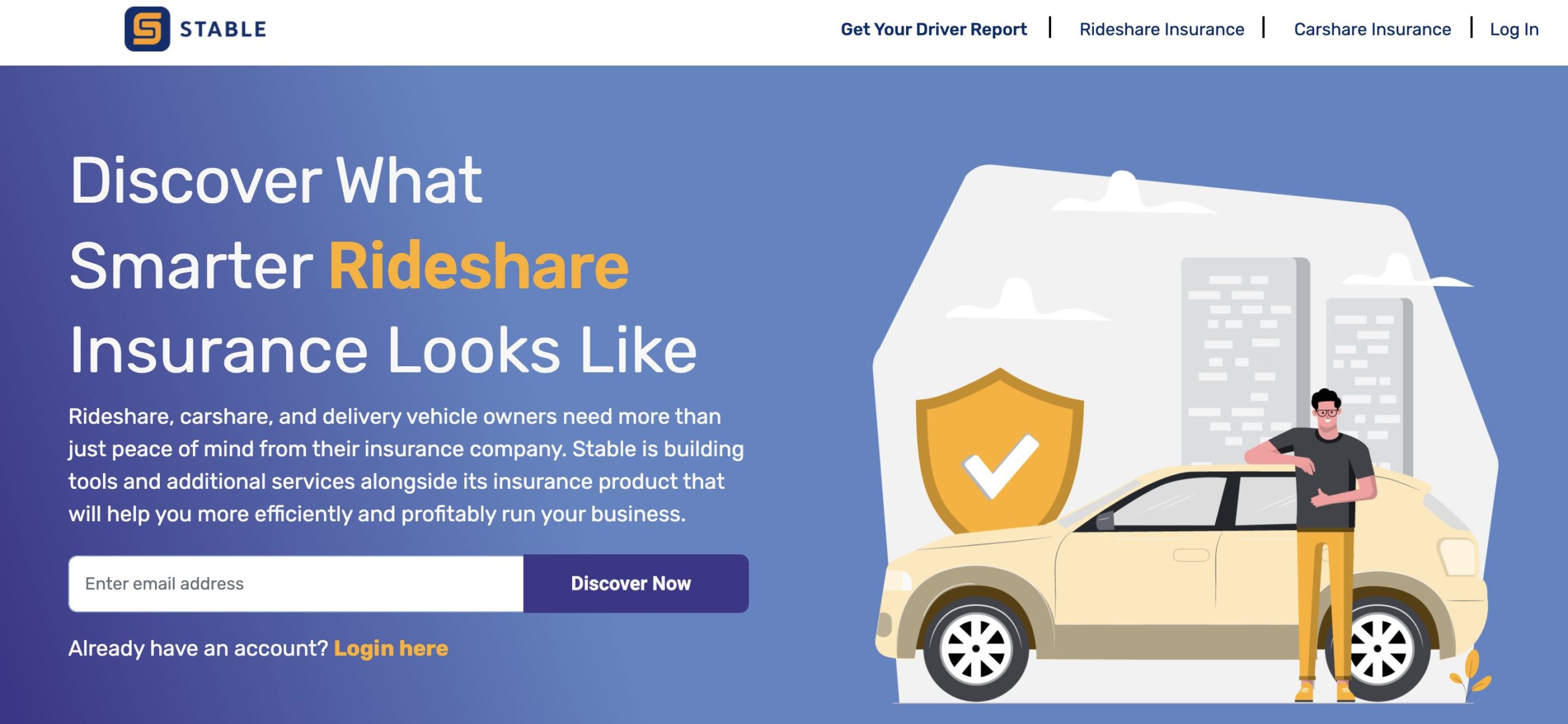This is a cropped screenshot of the Stable website's homepage.

In the top left corner, the Stable logo is prominently displayed with the word "Stable" written next to it in dark blue font. The logo itself features a black base with a yellow 'S' formed by two interlocking half boxes or U-shapes.

Navigation links are aligned horizontally near the logo: "Get Your Driver Report," "Rideshare Insurance," and "Carshare Insurance" are all hyperlinked in blue. The "Log In" link is also included in this menu.

The webpage's body has a blue background. Visible at the top left of the page is the headline "Discover what smarter rideshare insurance looks like," where the word "Rideshare" appears in orange while the rest of the text is in white. Below this header is a paragraph written in smaller white text.

Towards the bottom left of the page, there's an input box labeled "Enter email address." To its right is a blue button with the text "Discover Now." Just below this input box, there is a prompt that reads "Already have an account? Log in here," with the "Log in here" text highlighted in gold or yellow.

On the right side of the webpage, there is a grayscale clipart image of tall skyscrapers as a backdrop. Overlaid on this is a colorful car with a man standing beside it, wearing yellow pants and a black shirt. To the right of this image, a shield icon with a white checkmark symbol is present, emphasizing security or protection.

This detailed layout captures the essence of the Stable website's homepage, highlighting both navigational elements and visual aesthetics.